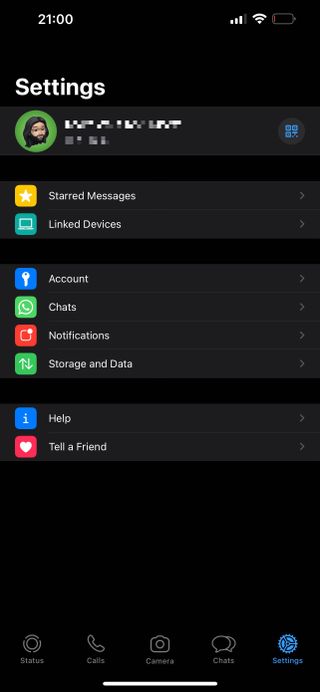This is a detailed description of a screenshot taken from a smartphone. The image is portrait-oriented and rectangular, with a height approximately two and a half to three times its width. The background is predominantly black.

At the top of the screenshot, in white font, the time is displayed as 21:00 hours. Adjacent to the time is a network status icon showing three out of four bars, a full Wi-Fi meter, and a battery icon. The battery icon is horizontal with a black background and a red meter, indicating that the battery is nearly depleted.

Below the status bar, there is a white header labeled "Settings." Beneath this header, a gray rectangular box spans the width of the screen, containing an avatar. The avatar is enclosed within a green circle and depicts a man with long hair. Text near the avatar is blurred for privacy. 

Centrally positioned on the screen is a blue icon resembling a game controller, set against a gray circular background. 

Following this are two gray boxes, laid out horizontally, labeled "Start Messages" and "Link Devices." 

Beneath these, four equally sized gray boxes stretch horizontally across the screen. These boxes are labeled "Account," "Chats," "Notifications," and "Storage and Data," each accompanied by an icon on the left.

Towards the bottom of the image, there are two more gray boxes labeled "Help" and "Tell a Friend."

Finally, aligning the bottom edge of the screenshot are options for navigation: "Status," "Calls," "Camera," "Chats," and "Settings." The Settings option is marked with a gear icon and is highlighted in blue.